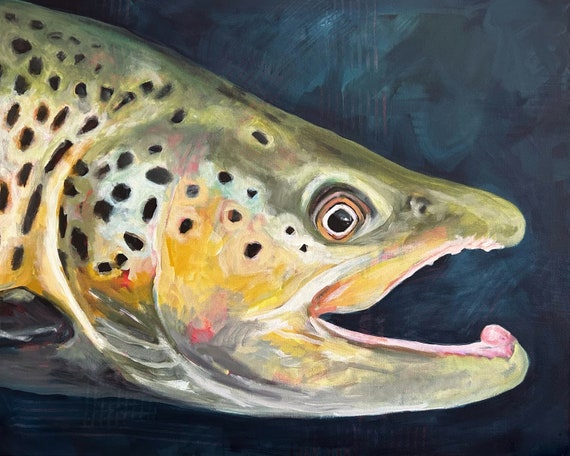The image depicts a detailed painting of a fish head, which exhibits characteristics that could resemble both an eel and a salmon. The fish has a long, eel-like head featuring a prominent, V-shaped mouth with big jaws, suggesting a predatory nature. The mouth is open, revealing a pink interior, although no teeth are visible. The body, partially shown, is primarily green with black spots, and there are yellow hues interspersed within the green areas, particularly around the middle of the body. Notably, the fish also exhibits dark spots, especially around the gills and the upper part of its body. The eyes have black pupils surrounded by white and more prominently by yellow. The background of the painting stands out as a dark, cobalt blue, adding a stark contrast to the fish’s vibrant colors and creating a sense of depth despite the somewhat smudgy, whimsical portrayal of the underwater scene.